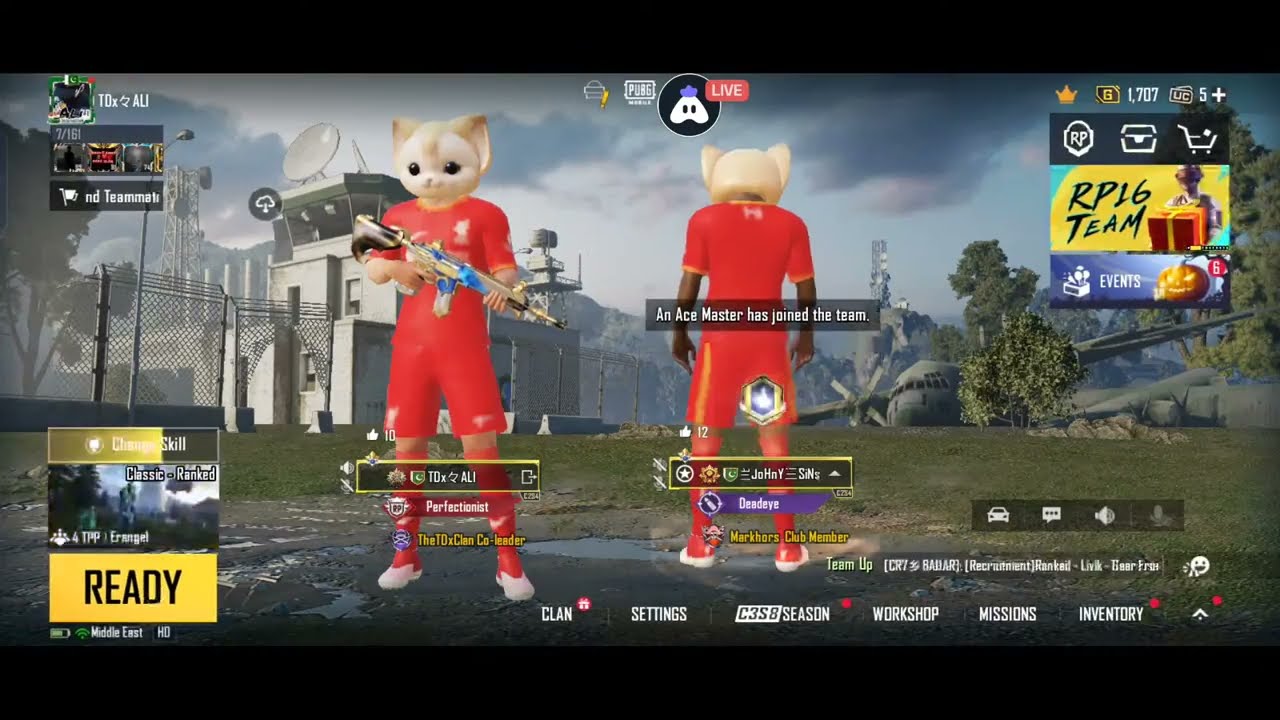The image depicts a waiting screen from a video game, indicated by long black bars at the top and bottom of the screen. The background showcases a realistic outdoor setting with grass, trees, overcast clouds, a fallen green cargo plane, and a building with a broken, tall barbed wire fence, suggesting it might be a prison.

Two characters occupy the foreground. Both are dressed in red soccer jerseys and shorts, red knee pads or shin guards, and white footwear. Their most striking feature is their large, cat-like helmets with giant ears, which contrast sharply with the otherwise gritty environment. The character on the left faces forward, brandishing a gold and blue assault rifle, and has white arms. The character on the right, seen from the back, has black arms but is similarly dressed.

Above the characters, "An Ace Master has joined the team" is displayed, potentially referring to the player's title or status. In the upper right corner, "RP-16 team" is highlighted, adjacent to icons like a treasure chest, a shopping cart, and a gift box. Below these icons, "events" is marked with a pumpkin face, suggesting a Halloween theme. Other text is visible, such as "clan settings," "C3, S3," "Season," "Workshop," "Mission," and "Inventory," with red stars beside specific terms.

An intricate overlay includes elements like a crown, a yellow paper with "1707" on it, and a bag marked with "5+" on the right. The bottom left displays a white box with the word "Ready," indicating the game awaits the player's action.